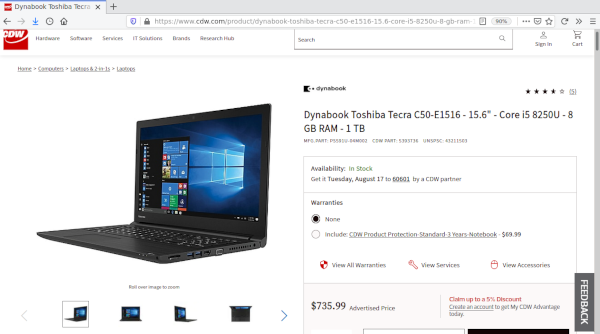The image depicts a user shopping for a laptop on the CDW website (www.cdw.com). The screen shows the Toshiba Dynabook Tecra C50-E1516-15.6” laptop, featuring a Core i5-8520U processor and 8GB of RAM. Specific details such as the part number, COM part, and UNSPSC number are displayed but are small and hard to read. The laptop is in stock and estimated to arrive by Tuesday, August 17th to ZIP code 50501 via a CDW partner. 

In the warranty section, the default option selected is “None,” with the alternative being “CDW Product Protection Standard 3 Years Notebook” for $69.99. A shield icon labeled “View All Warranties” appears, along with a red wrench icon for “View Services” and a red mouse icon for “View Accessories.” The advertised price of the laptop is $735.99, with an option to claim up to a 5% discount. To access this discount, the user is prompted to create an account for CDW Advantage.

The page includes customer feedback with the Toshiba Dynabook rated at four stars based on five reviews. The CDW logo, a red box with “CDW” written in white and a white line extending from beneath the "C" past the "W" and out of the box, is prominently displayed. The user appears to be browsing the site using the Edge browser, evident from the typical browser features, along with visible sign-in and cart buttons.